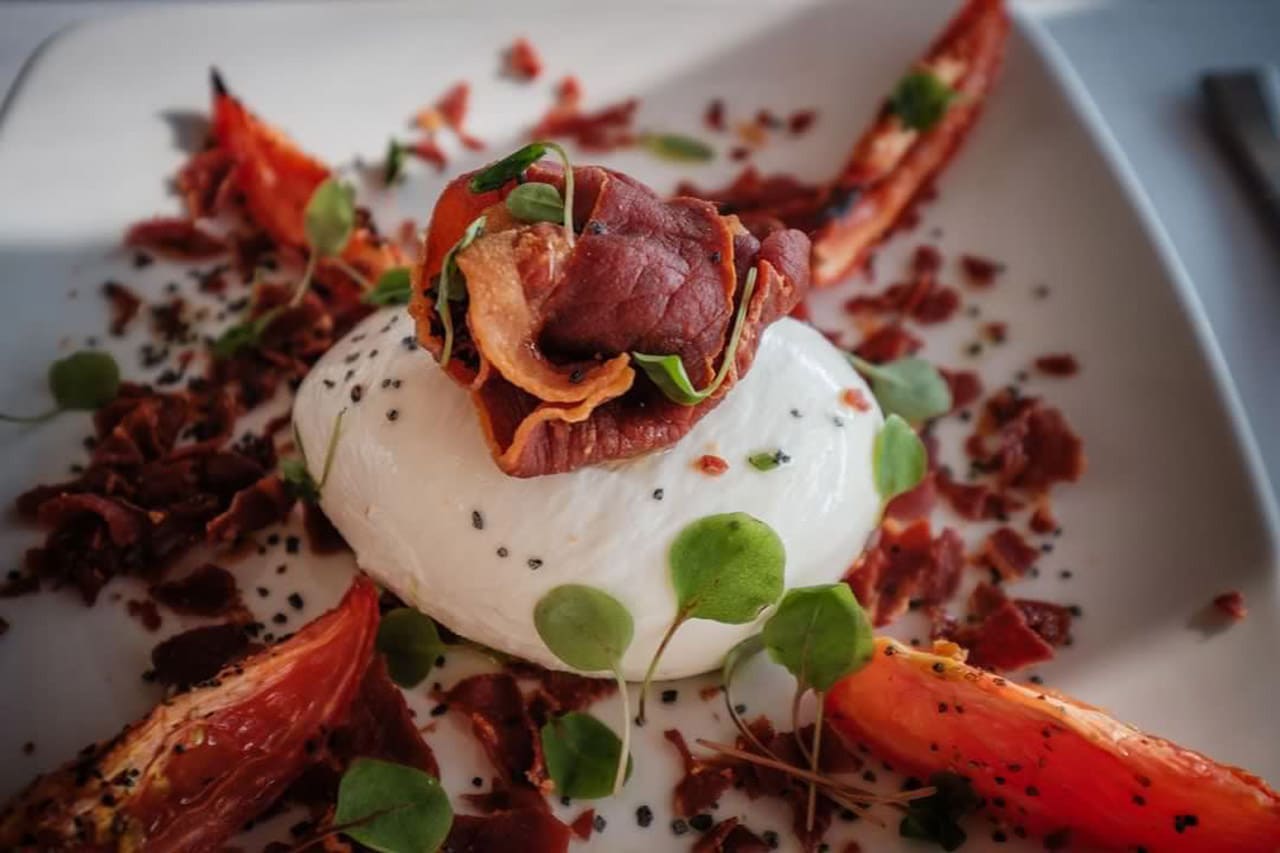This image showcases a gourmet dish, likely served at a high-end restaurant, presented on a round white ceramic plate placed on a white tablecloth, with a utensil to the right. The dish features a large dollop of a creamy, white cheese or sour cream-like substance in the center, speckled with black pepper. Atop this, there's a rolled piece of either raw or poached fish, possibly bacon, garnished with a scattering of herbs and microgreens. Surrounding the central dollop, arranged in a square formation, are four pieces of red pepper, lightly cooked, extending outwards. Additionally, there are sprinkles of crumbled meat, likely bacon bits, around the plate, which also has a noticeable shadow cast over it. This intricate arrangement of reds, greens, and whites makes the dish not only a culinary delight but a feast for the eyes.